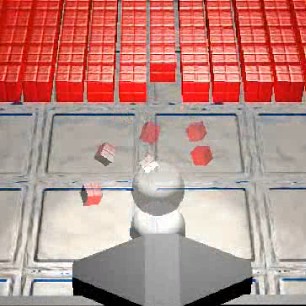The image features a collection of red cubes stacked at the top, each composed of four smaller cubes. The ground is a meticulous grid with green and blue divisions set against a predominantly gray surface. At the center of the ground, two prominent spheres are positioned, one above the other. Another focal point is an intricate eight-sided shape with distinctively elongated diagonal sides and flat edges oriented towards the north, south, east, and west. The overall backdrop is an expansive, predominantly white cubic ground, extending into the distance.